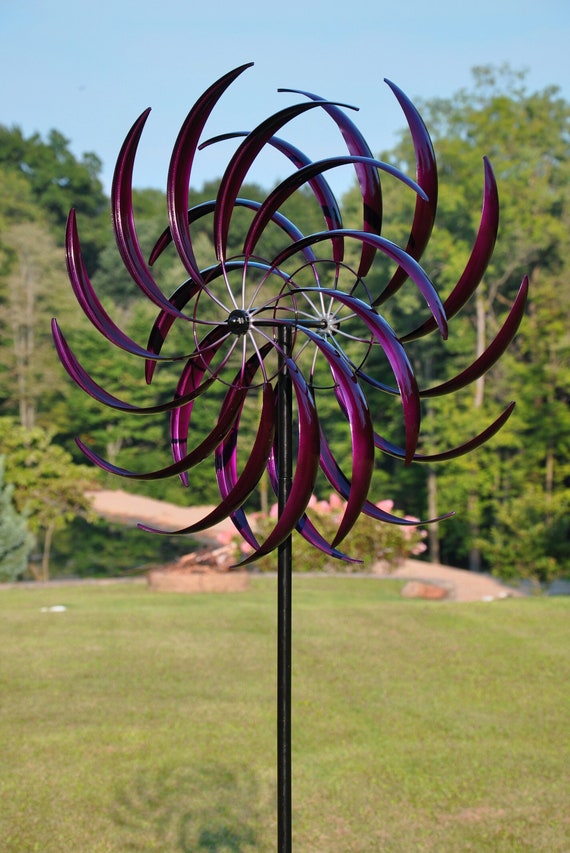The image showcases an intricate, metallic wind spinner yard decoration composed of dark maroon and iridescent purple metal spokes resembling feathers. The sculpture is mounted on a black pole staked into a lush green yard. The wind spinner features two sets of 14 spiky blades, curving upwards and arranged in a mirrored fashion, designed to catch the wind and spin gracefully. The background presents a vivid landscape with a blue sky, verdant green trees, and an expansive grassy field. Additionally, there’s a pink flowering bush and a somewhat blurry pathway leading into a canopy of trees, giving the scene a surreal, almost AI-generated feel. The artistic design and the natural surroundings combine to create a visually captivating and serene outdoor scene.